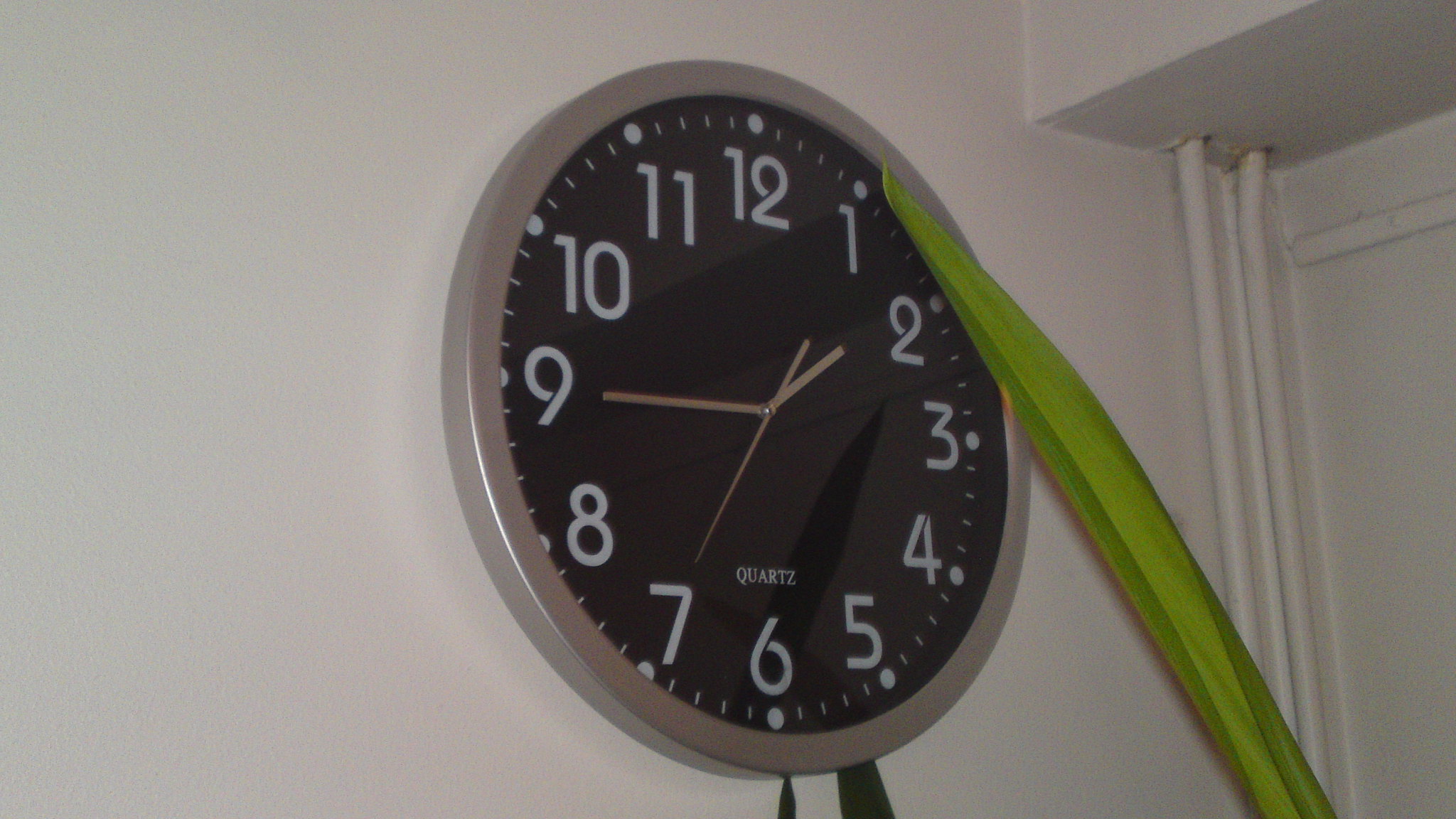The image depicts a sleek, contemporary wall clock positioned near the ceiling at the corner of a white wall. The clock, which is circular in shape, has a stylish silver-toned metal rim and a sophisticated black face. Prominently displayed on the black face are white numerals and dots marking the hours, complemented by silver hands. The word "QUARTZ" is inscribed in white just above the six o'clock position.

In the foreground, a long, slender plant leaf with a pointed tip is partially covering the right side of the clock, its tip precisely aligning with the number one. The leaf extends up the wall, subtly touching the clock face between the numbers one and two. Additionally, a smaller section of another leaf from the same plant peeks out below the clock, near the numbers five and six. In the right-hand corner of the image, two wires, painted white to blend seamlessly with the wall, run vertically underneath a ledge, adding an understated, utilitarian detail to the scene.